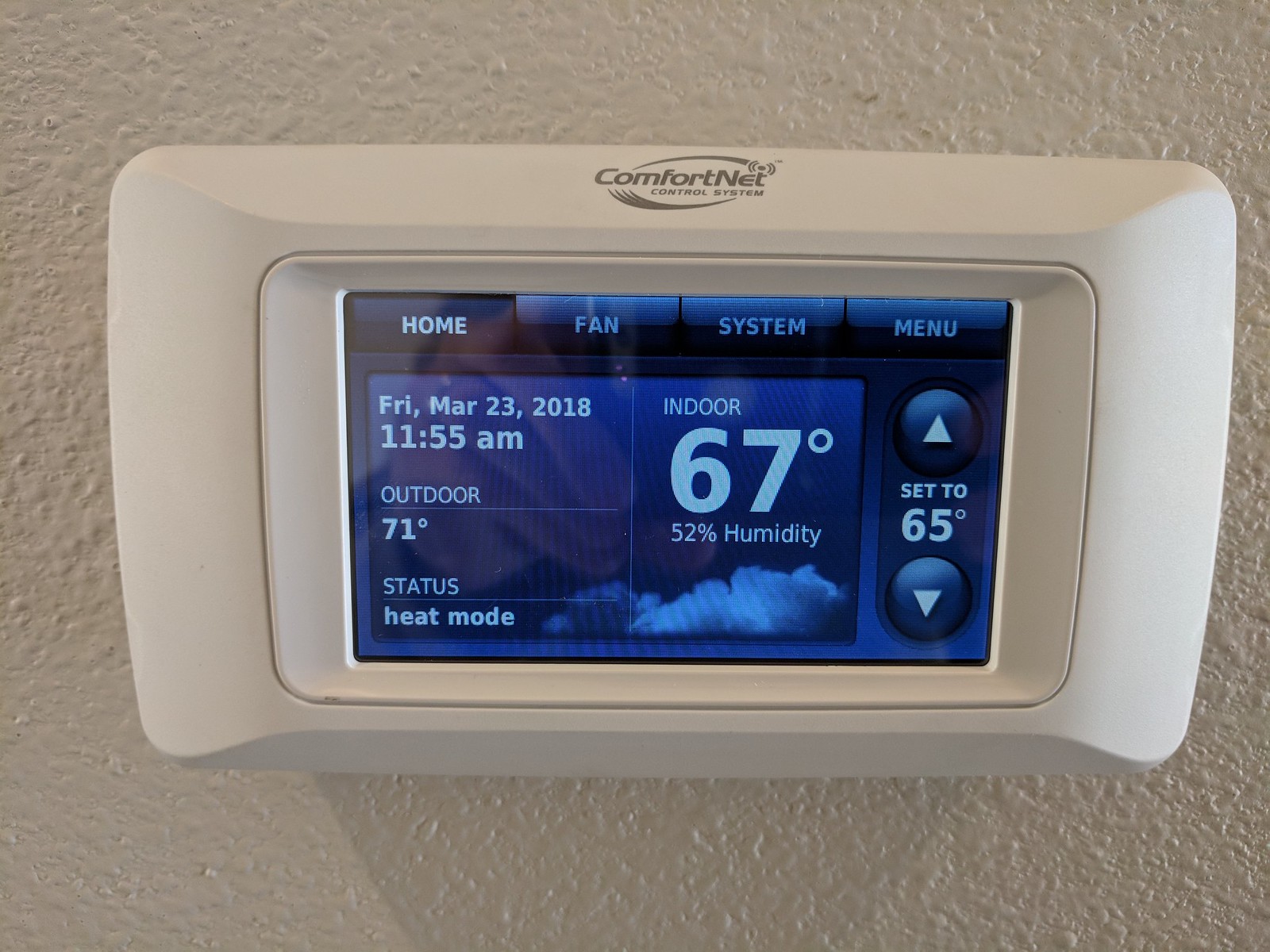This is a detailed color photograph of a Comfortnet Control System thermostat. The brand name is prominently displayed at the top center of the device. The screen is currently on the "Home" tab, with additional navigation options for "Fan," "System," and "Menu" displayed at the top of the interface. The current date and time are shown as Friday, March 23rd, 2018 at 11:55 a.m. 

The thermostat indicates that the outdoor temperature is 71°F, and the system is currently in "Heat Mode." To the right, the indoor temperature is noted as 67°F with a humidity level of 52%. At the bottom right corner of the screen, there is a small cloud icon, possibly serving as a weather indicator. 

Adjacent to this, there are two triangular buttons for temperature adjustment - an upward-pointing arrow for increasing the temperature and a downward-pointing arrow for decreasing it. The thermostat is set to maintain a temperature of 65°F, as displayed in the center of the screen.

The device is mounted on a white, slightly textured wall, reminiscent of a popcorn ceiling finish. A shadow is cast by the thermostat towards the bottom right, adding depth to the image.